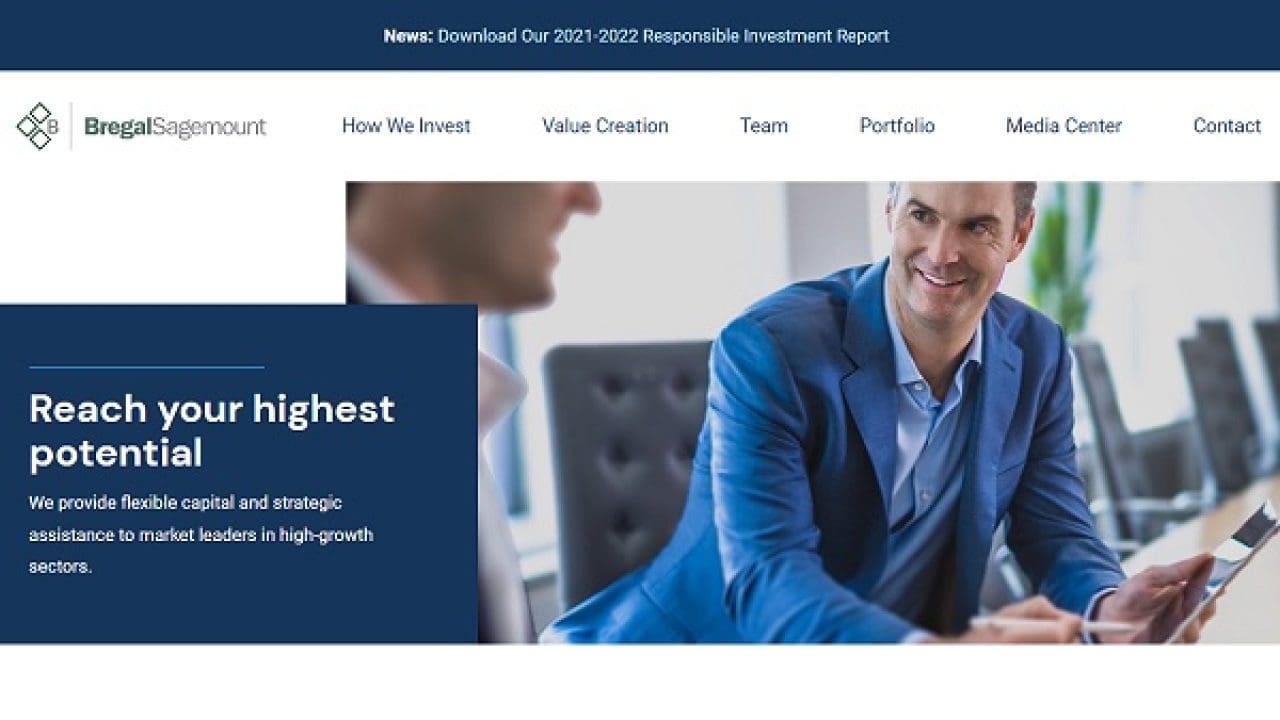The Bregel Sagemount homepage features a comprehensive layout dedicated to their investment strategies and team. 

On the left, the Bregel Sagemount icon is prominently displayed, consisting of three diamonds arranged as an arrow pointing left, followed by the letter "B." The page offers navigation options including news updates, access to their 2021-2022 Responsible Investment Report, information on their investment philosophy, value creation strategies, team details, portfolio insights, media center, and contact information. A motivational tagline, "Reach your highest potential," underscores their commitment to providing flexible capital and strategic assistance to market leaders in high-growth sectors.

Dominating the page is a large, vivid image capturing a moment of professional interaction. A fair-skinned gentleman, dressed in a blue blazer and light blue shirt open at the collar, sits in a black office chair, smiling warmly. His short, grayish-black hair frames a friendly but attentive expression as he engages with another fair-skinned gentleman. The second individual, though slightly blurred, appears to be in a lively conversation with the first. Seated at a long meeting table adorned with additional chairs, the man in the blazer holds either a stylus or pen, pointing towards a tablet, suggesting an active discussion or presentation in progress.